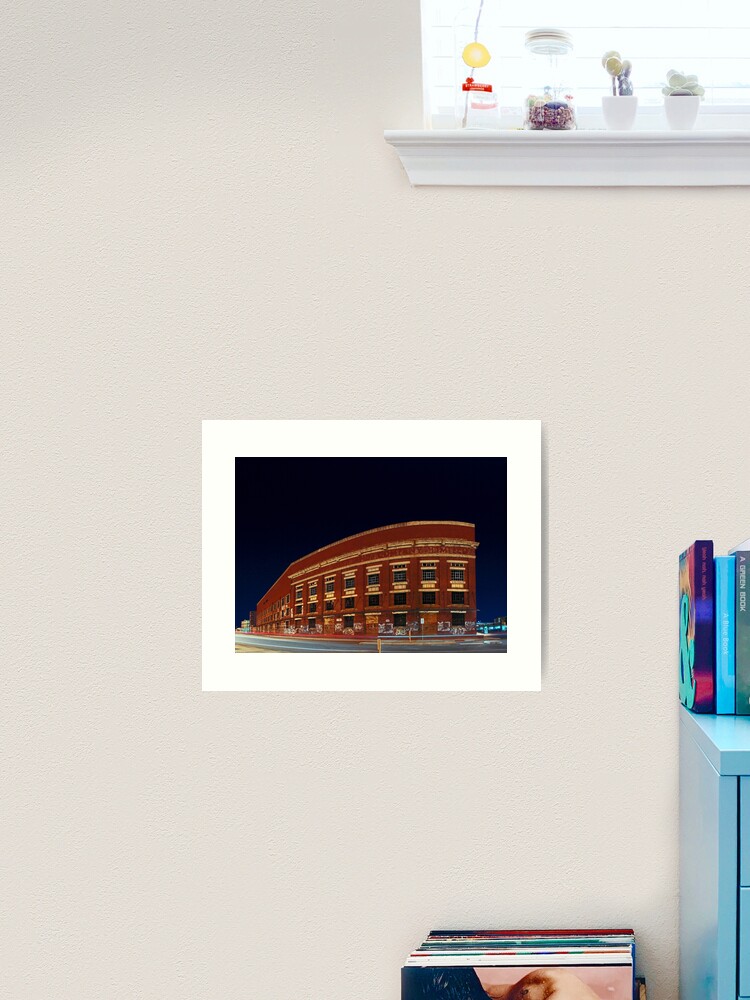The image displays a detailed interior scene centered around a framed photograph of a three-story brown brick building, possibly located in an urban area like Philadelphia. The building, characterized by yellow trimming around its black windows, stands against a dark, nighttime sky with a grey street running horizontally in front of it. This photograph is set within a white matte border and is mounted on an off-white or cream-colored wall.

To the upper right of the framed picture is a white windowsill adorned with various tchotchkes. Among these are a see-through glass jar, which could be a mason jar, some white ceramic cups containing small potted plants, and possibly a succulents.

In the bottom right quadrant of the image, there is a teal blue metal desk or filing cabinet. Positioned on top of the desk are several vertically arranged books, including dark blue, light blue, and green volumes. Below the desk, at the edge of the frame, lies a collection of books or vinyl records stacked in a manner that only their spines are visible.

The scene creates a cozy and eclectic vignette, combining art, plants, and books to evoke a well-lived, personalized space.